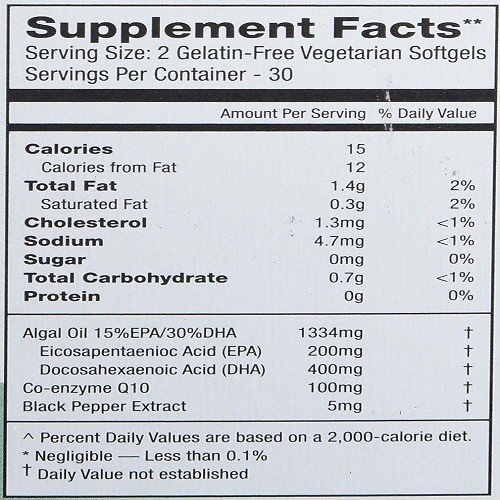Close-up image of a detailed nutritional facts label for a food product. The label is presented on a white rectangular background with black borders, utilizing a mix of bold and unbolded black font. The title "Supplement Facts" is displayed prominently at the top. Below, it specifies the serving size as "two gelatin-free vegetarian soft gels" and indicates that there are 30 servings per container. The label methodically lists various nutritional categories including calories, total fat, cholesterol, sodium, sugar, carbohydrates, and protein. For each category, it provides precise amounts per serving in milligrams (mg), grams (g), and the corresponding percentages of the daily value.